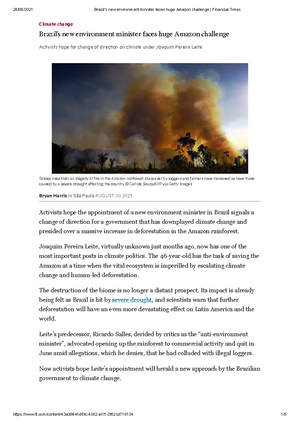This image captures a digital article discussing Brazil's new Environment Minister and the significant challenges he faces regarding the Amazon Rainforest and climate change. At the top of the article, the phrase "Climate Change" stands out in red letters. Below this headline, there's a subheading in smaller print that reads: "Activists hope for a change of direction on climate under Joaquim Pereira Leite." 

Dated August 20, 2021, the article is structured into five distinct paragraphs, providing detailed insights into the situation. In the middle of the page, there is an interactive element labeled "severe drought" in a teal color, indicating that readers can click on it for further information. 

The upper section of the article features a striking image, presumably depicting the aftermath of forest fires. The photograph shows thick smoke in shades of brown, orange, and yellow billowing up from a forested area, with visible plants on the ground, possibly indicating a section of rainforest.

The article concludes with small print details at the very bottom, further emphasizing the pressing urgency of climate action and environmental protection in Brazil.